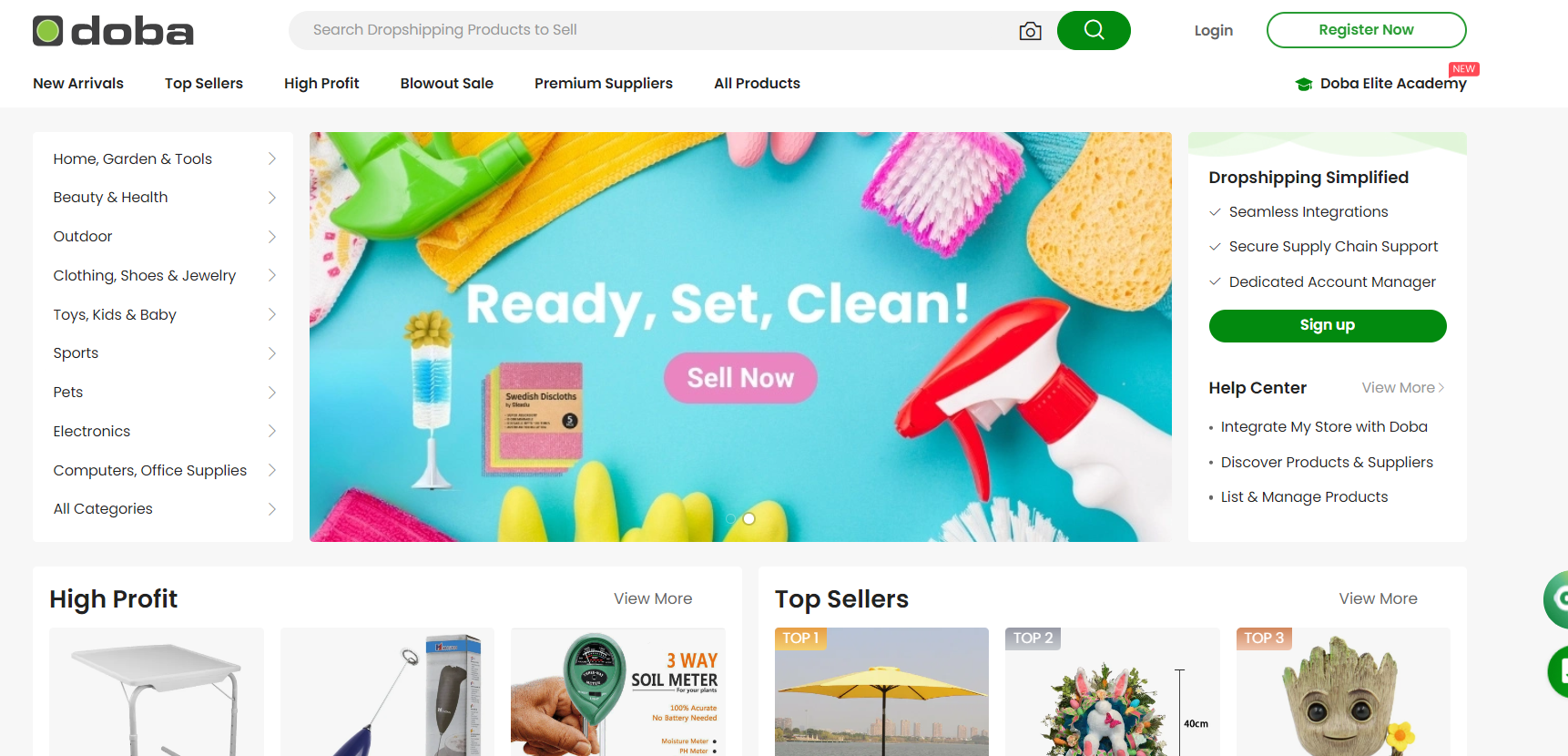This image comes from the website DOBA, an e-commerce platform for dropshipping products. The header features a search bar labeled "Search drop shipping products to sell," accompanied by a camera icon on its right side, indicating an option to perform a visual search. The search bar also contains a green area with a white magnifying glass icon, signifying the search function. 

At the top-left of the page, there are navigation options labeled "New Arrivals," "Top Sellers," "High Profit," "Blowout Sales," "Premium Suppliers," and "All Products," allowing users to explore product categories efficiently. 

The central part of the image showcases an assortment of cleaning items, including a spray bottle, sponge, scrubber, gloves, bottle washer, and Swedish dishcloths, arranged in a circular pattern around the words "Ready, Set, Clean". Below this, there's a pink "Sell Now" button, indicating an actionable step for users. The background for this section is a vibrant teal color, making the products and message stand out.

Additionally, there's a section highlighting "High Profit" and "Top Seller" items, and a green "Sign Up" button located at the upper-right corner of the webpage, inviting new users to join the platform.